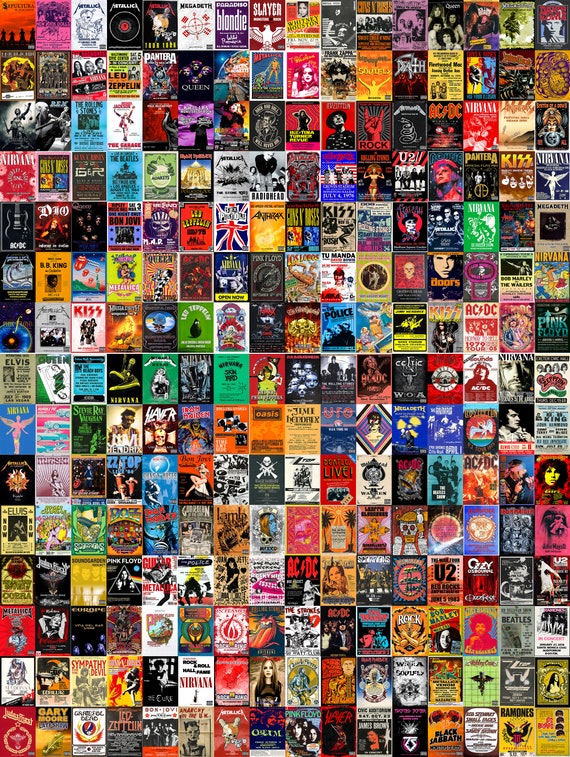This image is an intricate and vibrant collage of rock and metal band posters, featuring an eclectic mix from iconic groups like Nirvana, Kiss, The Doors, ACDC, Black Sabbath, and Pantera, to legendary acts such as Led Zeppelin, Jimi Hendrix, The Beatles, Slayer, Iron Maiden, and U2. With approximately 140 to over 200 posters, this crowded and colorful assembly navigates through a multi-decade journey of rock history. The posters, arranged tightly in rows and columns, create a visually overwhelming experience that requires close inspection to identify each band. Prominent names like The Ramones, Elvis, Metallica, Queen, The Kinks, Megadeth, The Who, The Police, Cream, Pink Floyd, Bon Jovi, Dio, and Blondie further add to the nostalgia and diversity of the collection. The collage is a tall, narrow representation, roughly 12 posters high and 12 posters wide, each varying in design and color scheme yet collectively celebrating the dynamic spirit of rock and roll.